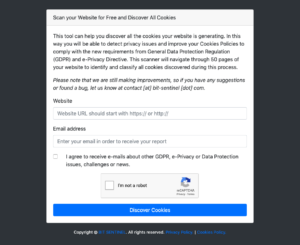The image depicts an intrusive pop-up notification on a website, urging users to utilize a free scanning tool to identify and analyze all cookies present on their site. The pop-up features a light gray box set against a dark background, making it clear that it is an overlay interrupting the main content.

The message within the pop-up explains that the tool will scan up to 50 pages of the user's website, identifying and classifying all cookies encountered. This helps webpage owners detect potential privacy issues and ensure compliance with evolving general data protection regulations and e-privacy directives.

The pop-up includes fields for entering an email address and the URL of the website to be scanned. Additionally, there is an option to agree to receive emails related to privacy, data protection issues, challenges, and news. To complete the form, users must check a box confirming they are not a robot and then click a blue "Discover Cookies" button to initiate the scan. A note at the bottom indicates that the developers are open to suggestions and bug reports, providing contact details for users to reach out.